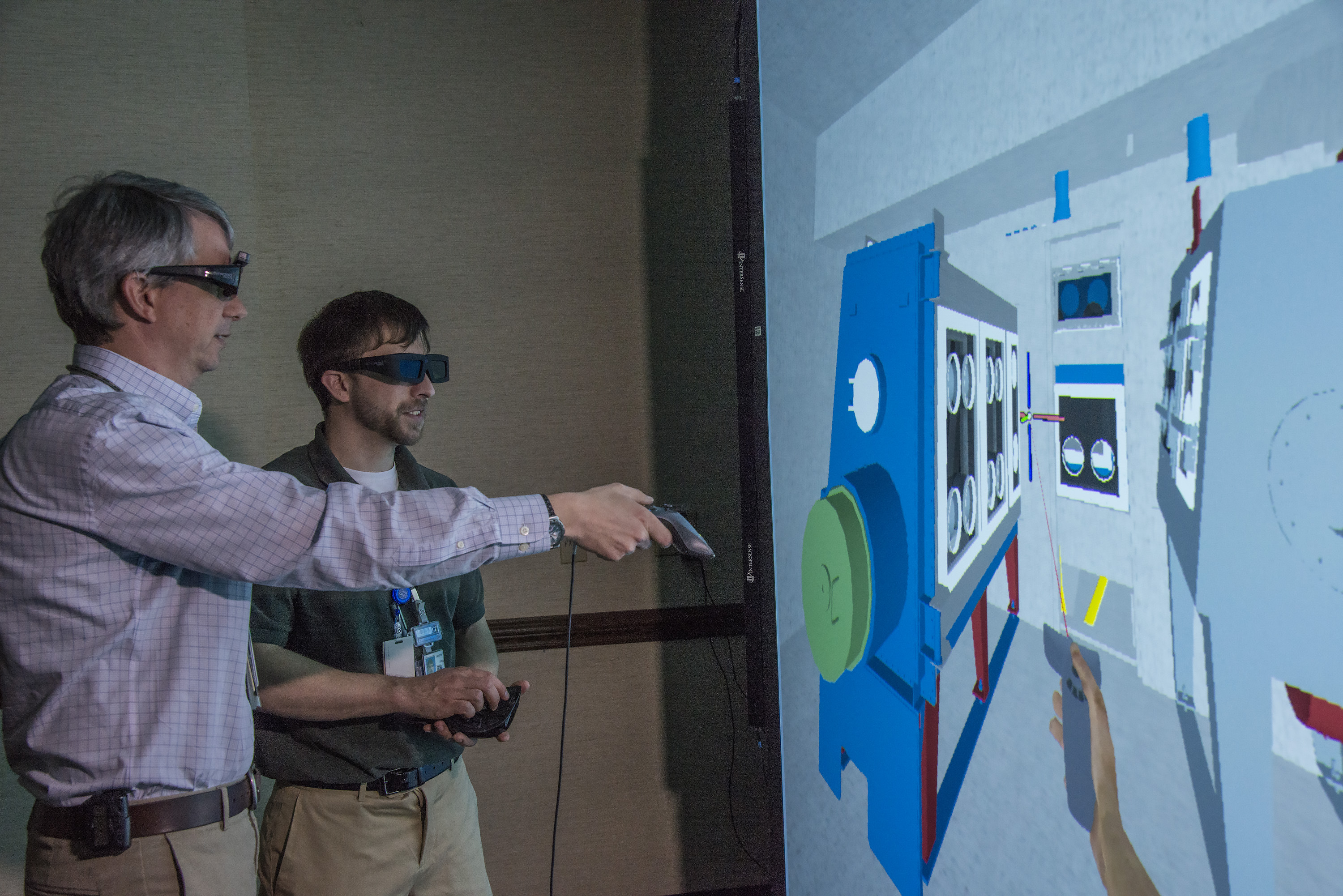This photograph captures two men standing in a room, engaged with a large screen displaying an illustration of a sizable, old-fashioned computer. Both men are wearing dark sunglasses. The older man, appearing to be in his fifties, has gray hair and is clean-shaven. He is dressed in a long-sleeved checkered shirt and tan pants, with a belt that has a pager attached. He holds a device resembling a video game controller in his right hand, which is connected by a cable, and points it towards the screen. The younger man, who has dark hair along with a mustache and beard, is wearing a short-sleeved polo shirt and tan pants. He also holds a device in his hand. Around his neck hang badges, possibly for access to different areas. They seem to be interacting with the screen, giving the impression that they are part of a virtual reality scenario. The room features bright, white walls with a green and blue design, enhancing the tech-centric atmosphere.